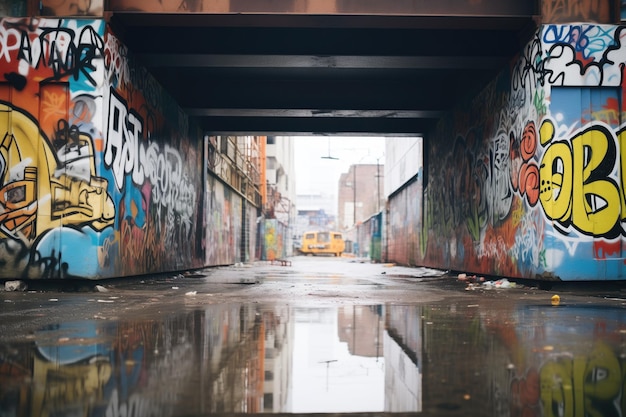A low-angle photograph captures an urban underpass, likely a bridge or tunnel, on a wet day with fresh rain puddles reflecting the scene. The ground appears to be brown asphalt or concrete, glistening with moisture. Concrete walls on either side are adorned with vivid graffiti, showcasing a mix of white, yellow, red, and blue backgrounds and an array of large, vibrant letters and artistic designs. The viewpoint narrows as it extends into the distance, where a yellow vehicle, possibly a car or bus, is discernible at the far end. In the background, blurred buildings and possible urban elements such as ladders are faintly visible, giving context to the urban surroundings and adding depth to the photograph.